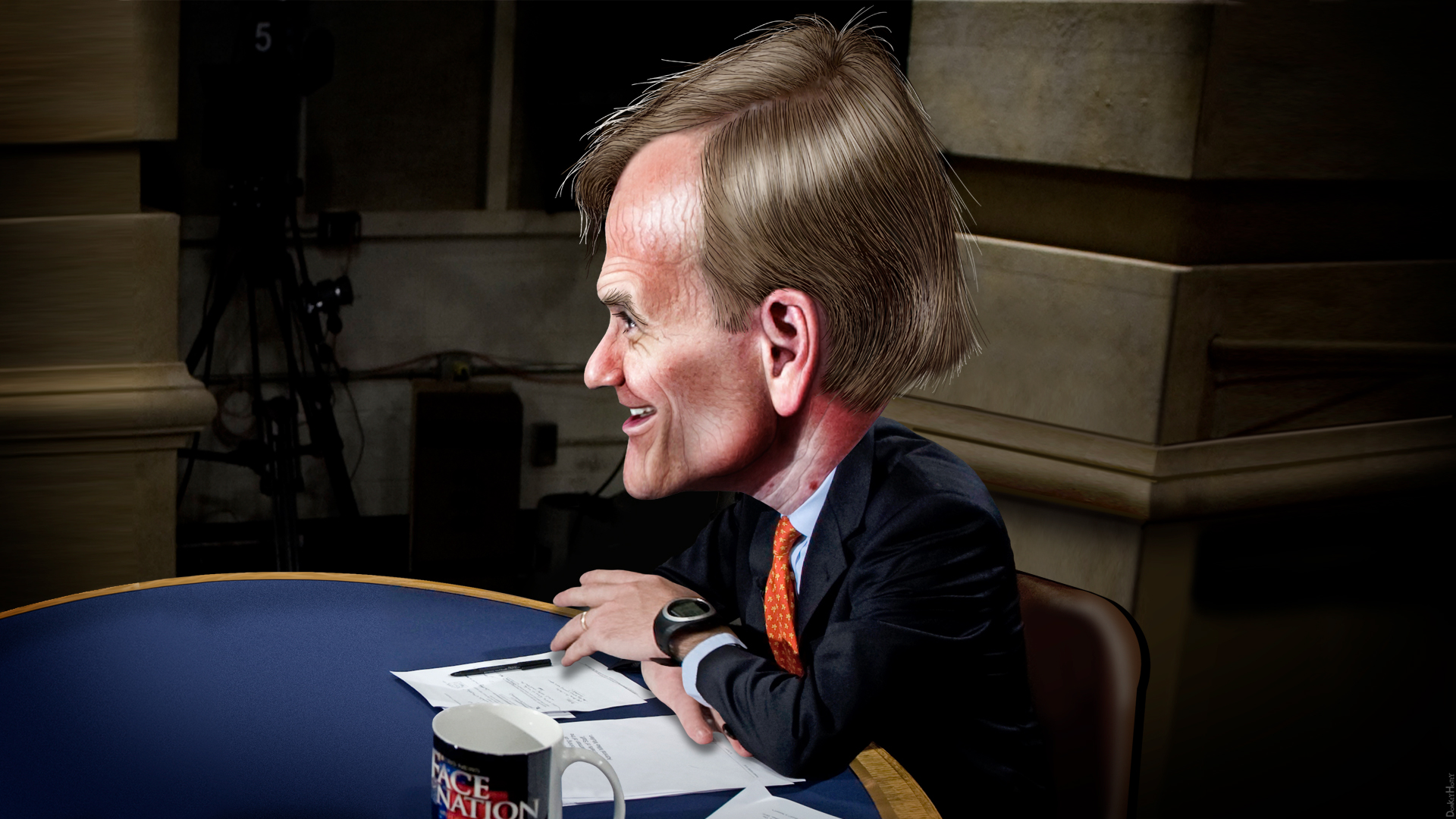The image depicts a highly stylized, exaggerated caricature of a man seated at a round table with a blue surface. The man's head is disproportionately large compared to his body, creating a cartoon-like effect. He is wearing a bluish-black suit jacket, a white button-up shirt, and an orange tie with yellow dots. His hands and ears are also exaggeratedly large. He is seated to the right of the table, looking towards the left, and resting his arms on some papers. In front of him sits a black coffee cup with "Face the Nation" printed on it, the inside of which is white. The backdrop behind him appears to be realistic, featuring a structure with heavy walls and pillars. He is seated on what seems to be a simple brown card table chair. The image combines elements of reality and animation, particularly in the exaggerated features of the man.